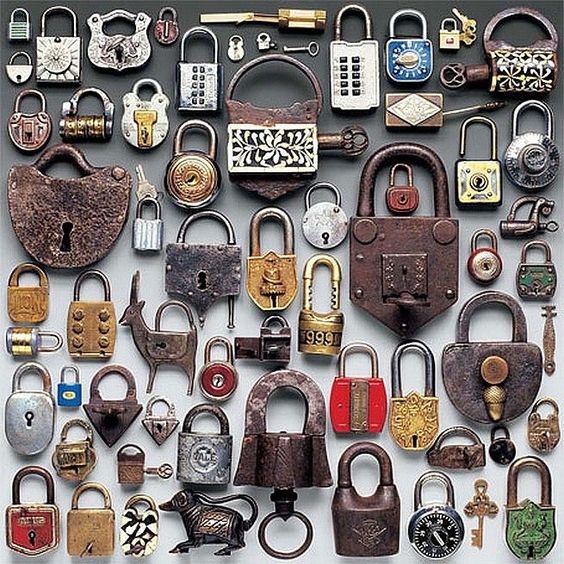The image is a detailed and vibrant color photograph featuring approximately 30 diverse locks arranged on a gradient gray background, transitioning from dark gray at the top to light gray at the bottom. These locks vary widely in style, size, and age, forming a fascinating array that spans both antique and modern designs.

Among the assortment, some locks are traditional, brass-colored, and fitted with skeleton keyholes, while others are sleek, modern apparatuses with push-button entry pads. Notably, there are several vintage locks exhibiting rust and weathering, suggesting significant age and usage. These include large, imposing padlocks with large shackles and old keyholes.

The photo also features a variety of whimsical and decorative locks. Notable examples include an animal-shaped lock resembling an antelope, a tiny lock no larger than a fingernail, a lock shaped like a purse, and a puppy-shaped lock located at the bottom left. Additionally, there is a blue rotary combination lock in the top right and a gold skeleton key at the bottom right. Some locks resemble small safes, akin to what one might find in a bank. 

While many of the locks operate with keys, a few employ combination mechanisms. The mix predominantly leans toward older, key-operated designs, highlighting a nostalgic collection that blends functional use with artistic expression. The combination of real-world realism and photographic representationalism lends the image a lifelike and detailed quality.